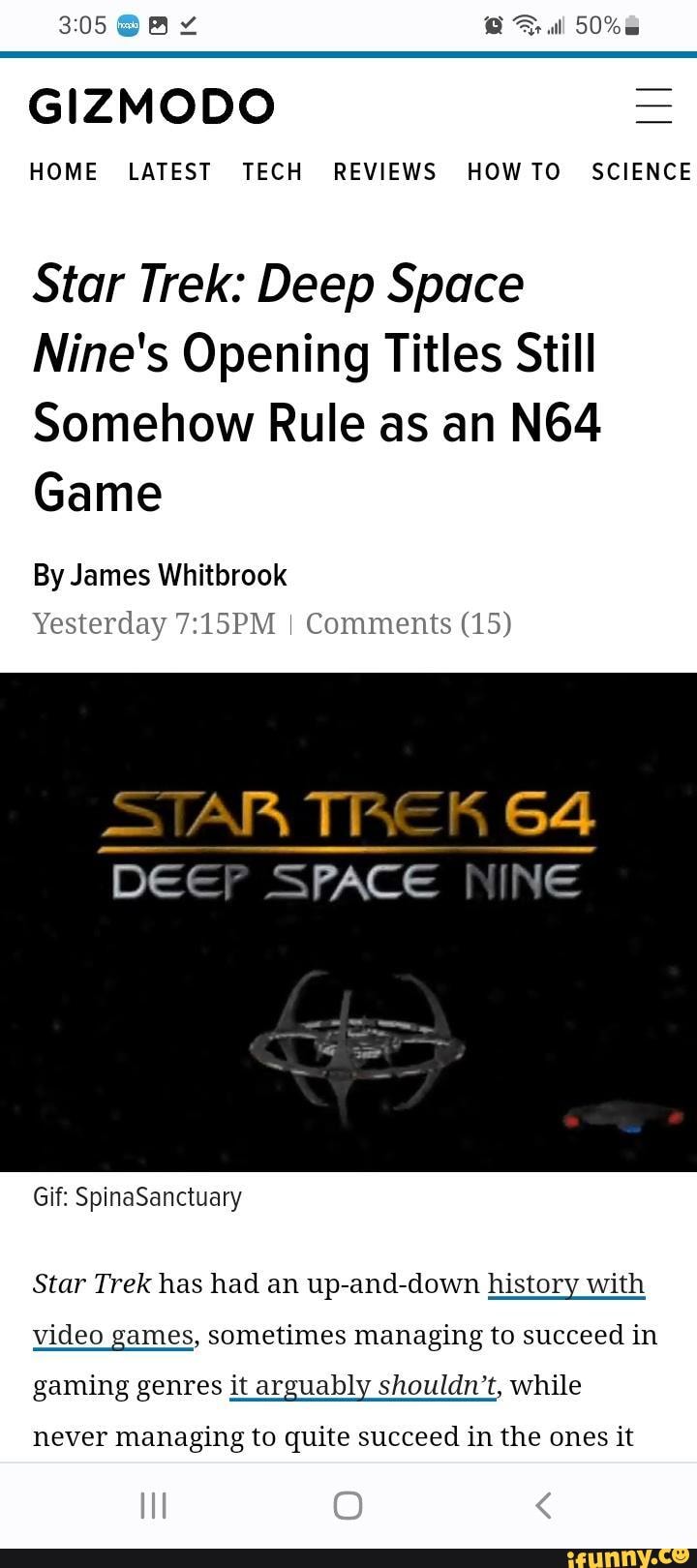Screenshot of a mobile device showcasing the Gizmodo app. The time displayed is 3:05, and the status bar shows a variety of icons including a blue notification icon, a photo icon, a checkmark, an alarm clock, Wi-Fi signal bars, cellular signal bars at 80%, and a battery icon at 50%. At the top left, there is a blue horizontal line with the text "Gizmodo" and a hamburger menu icon to the right. Below this, the navigation menu shows options: Home, Latest, Tech, Reviews, How-To, and Science.

The main article featured is titled "Star Trek: Deep Space Nine's opening titles still somehow rule as an N64 game," written by Jane Whitbrook and published yesterday at 7:15 PM, with 15 comments. The article's image includes a headline underlined with "Star Trek 64" and "Deep Space Nine" with a visual representation of a space station from the show, characterized by its iconic structural design of three hooks above and below, connected by a ring surrounding a central hub. Additionally, a spaceship is seen in the lower right heading towards the space station. A credit "GIF by Spinous Sanctuary" is visible beneath the image.

The introductory text of the article reads: "Star Trek has had an up and down history of video games, sometimes managing to succeed in gaming genres that arguably shouldn't, while never managing to quite succeed in the ones it..." Unfortunately, this text is cut off mid-sentence. The bottom of the screenshot shows parts of the navigation menu.